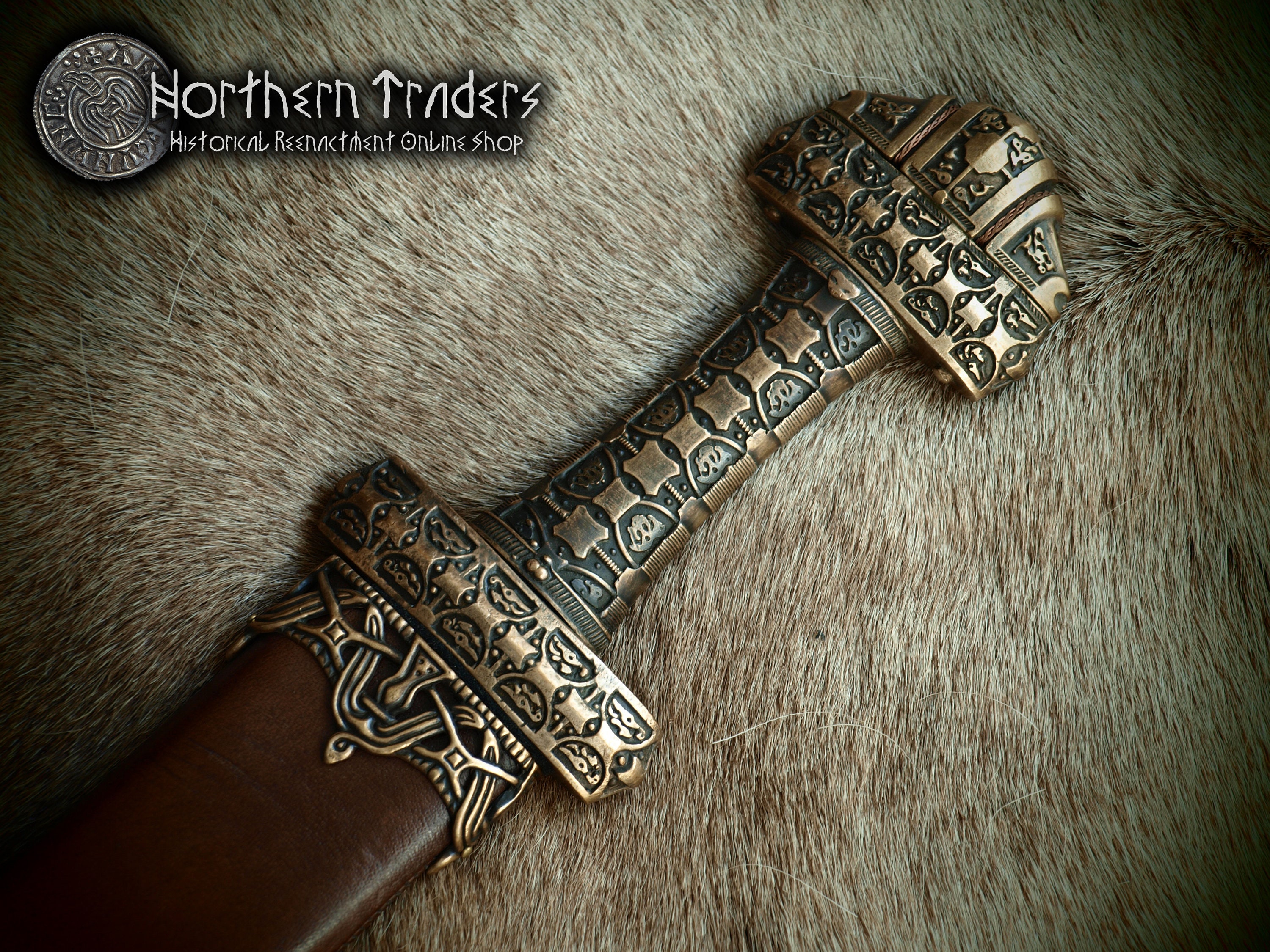The image showcases the ornate handle of a sword set against a background resembling animal fur, possibly wolf or deer hide, characterized by its light tan and brown shades. The highlight of the image is the intricately designed sword handle, crafted from a brass or bronzy gold-colored metal. The handle features detailed carvings, including a pattern of squares and a cap-like top with an elaborate design. The blade is partly visible, snugly encased in a brown leather scabbard. In the upper left corner, a round silver logo is present, next to the text "Northern Traders Historical Reenactment Online Shop" written in a rune-like font. The rich details of both the sword and the background create a compelling visual that speaks to historical craftsmanship.